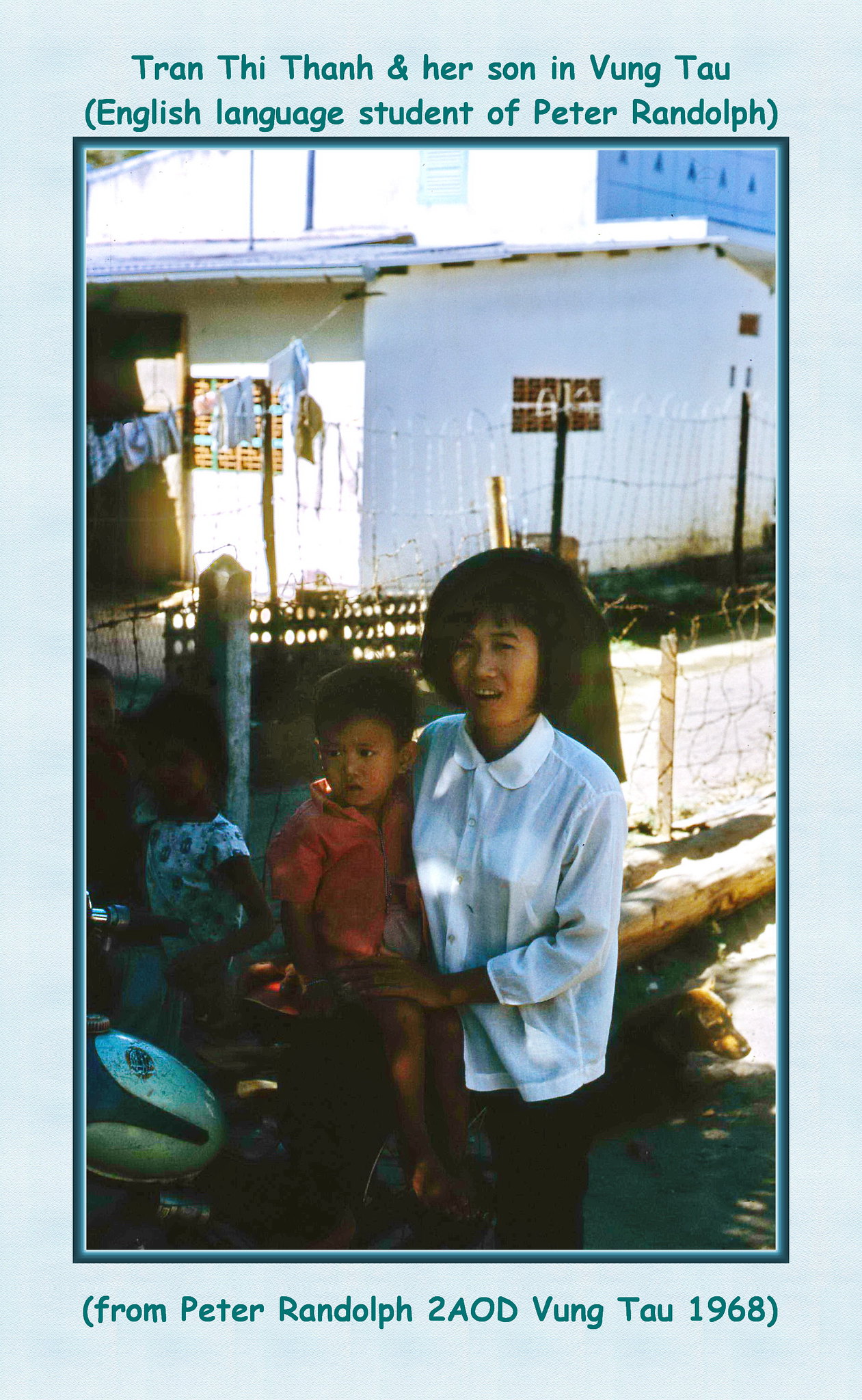The photograph is a poignant scene from the Vietnam War era, framed against a black background. It features a Southeast Asian woman with long, thick black hair styled in a bob, wearing a white button-up blouse and black pants. She stands in the center of the image, holding a young boy under her right arm. The boy, possibly two to three years old, is dressed in a light red button-up shirt, with short black hair. Nearby on the right, partially obscured by shadows, is another young child, likely a girl, looking up towards the woman. 

The background consists of a yard cluttered with various objects, suggesting a domestic setting. A white house or shop with a clothesline draped with clothes extends from a tree to the roof, lending the scene a lived-in feel. Behind the woman and children, a dirt road is visible.

At the top of the photo, it reads "Tran Thi Thanh and her son in Vung Tau," noting that Tran Thi Thanh was an English language student of Peter Randolph. The bottom caption states, "From Peter Randolph to AOOD, Vung Tau, 1968." The overall image is vertically rectangular, capturing the essence of a wartime domestic life intertwined with elements of ordinary existence.